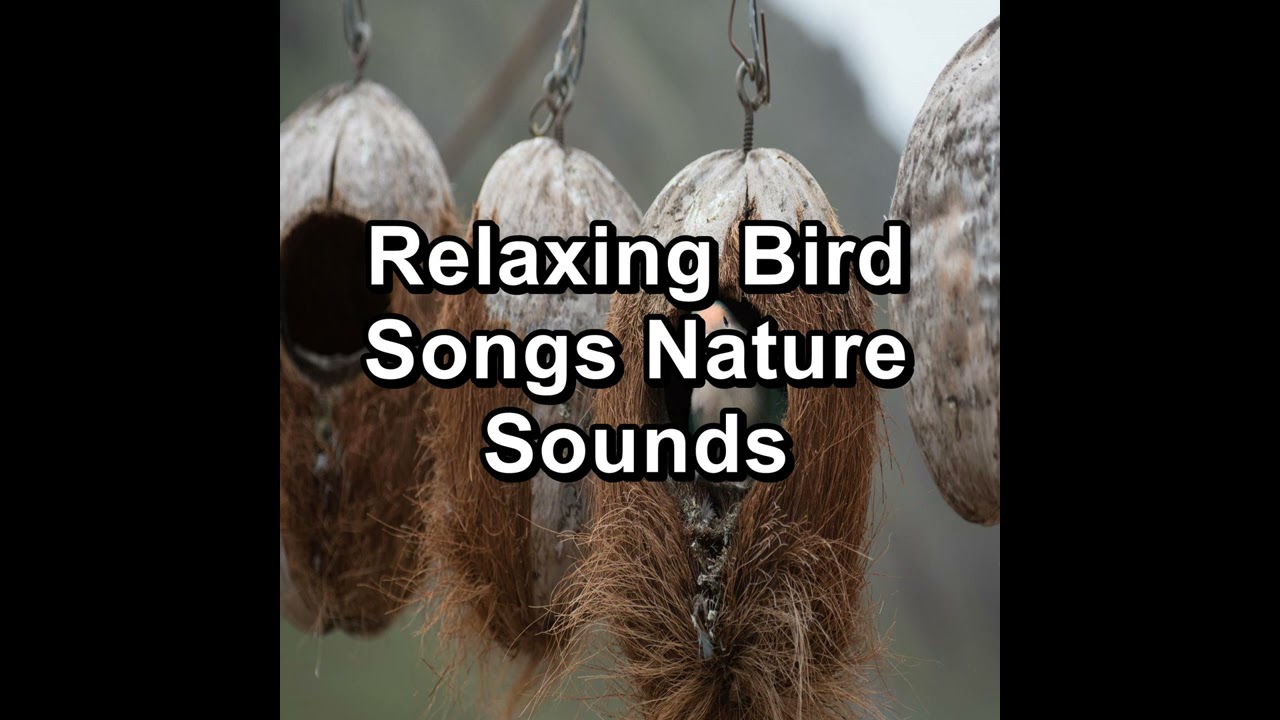The image features a central focus on four unique birdhouses that resemble elongated gourds or possibly coconuts, each with a wire hanging mechanism attached by screws at the top. The birdhouses are displayed against a blurry, indistinct backdrop, possibly resembling a mountainscape. The gourds are rough-hewn and brown with long plant fibers extending up the sides, while the tops are barren. Each birdhouse has a hollowed-out section in the middle, and one birdhouse shows a bird peeking out, though partially obscured by large, white bubble letters with a black outline that read "Relaxing Bird Songs, Nature Sounds." The image's composition is framed by thick black borders on the left and right sides, directing the viewer’s focus toward the center.